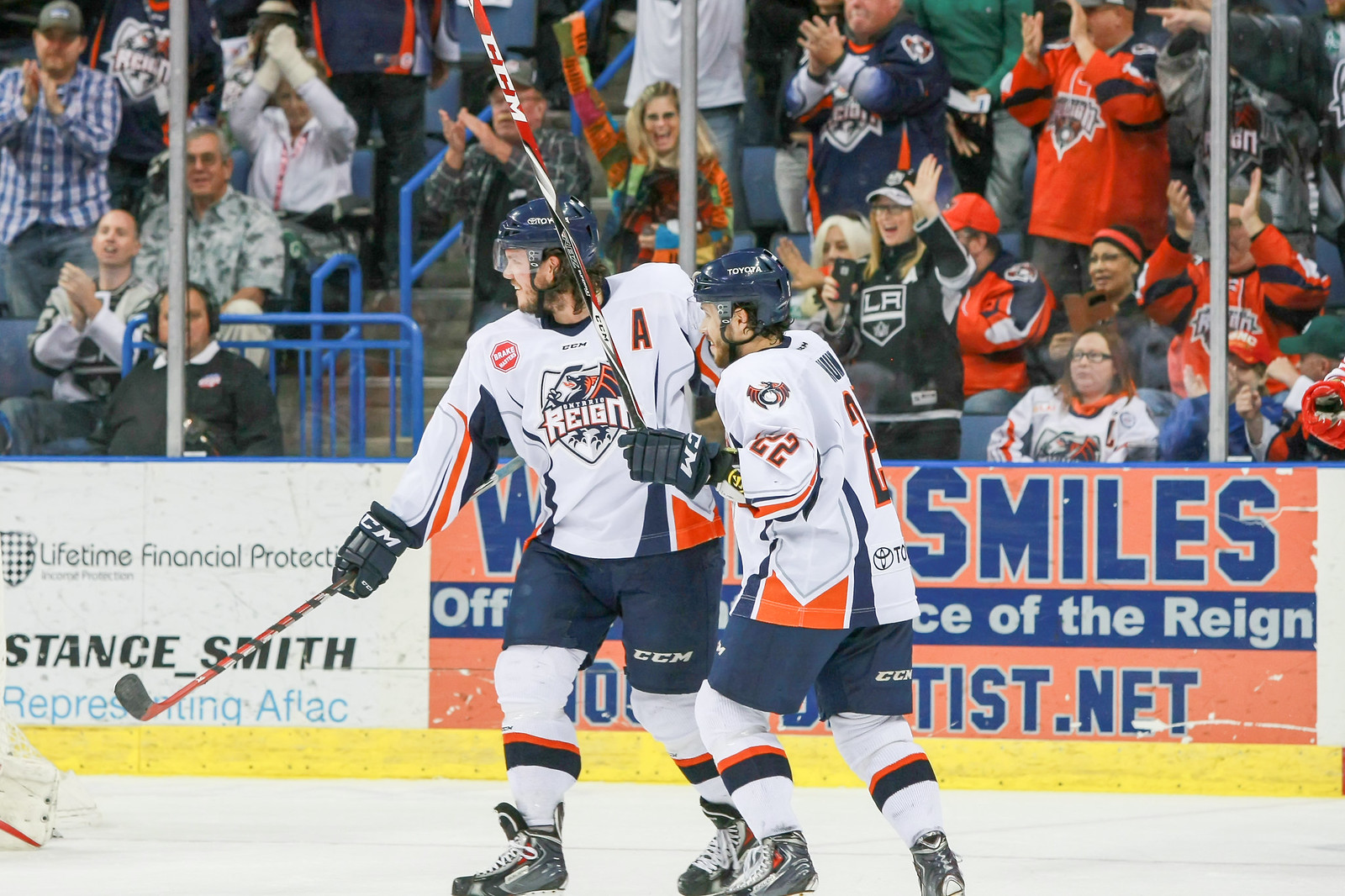In the image, we see a lively hockey game in progress featuring two players in action. Both players are clad in white jerseys with blue shorts and white trousers. The player on the left, identified by the letter "A" on his jersey, is skating from right to left with his hockey stick in his right hand. The jersey logo appears to spell "Reign". He is accompanied by another player on the right, who has his stick raised high, partially out of the frame, and bears the number 22 on his shoulder. Both players are equipped with full hockey gear, including helmets, gloves, and silver-gray ice skates.

The backdrop consists of sponsorship banners along the boards, with mentions of "Lifetime Financial Protection, Stan Smith representing AFLAC" and “Smiles Office of the Rain” along with an orange banner featuring "T-I-S-T dot net". Behind these boards, dozens of enthusiastic fans fill the stands. Some spectators are standing and cheering, notably a woman in her 20s with a baseball cap. Others can be seen sitting, including a woman donning the same jersey as the players on the ice. The seating area is divided by a staircase with blue railings on the left, leading to a busy section on the right where the fans are engrossed in the game. The visual captures the excitement and spirited ambiance of the live hockey event.